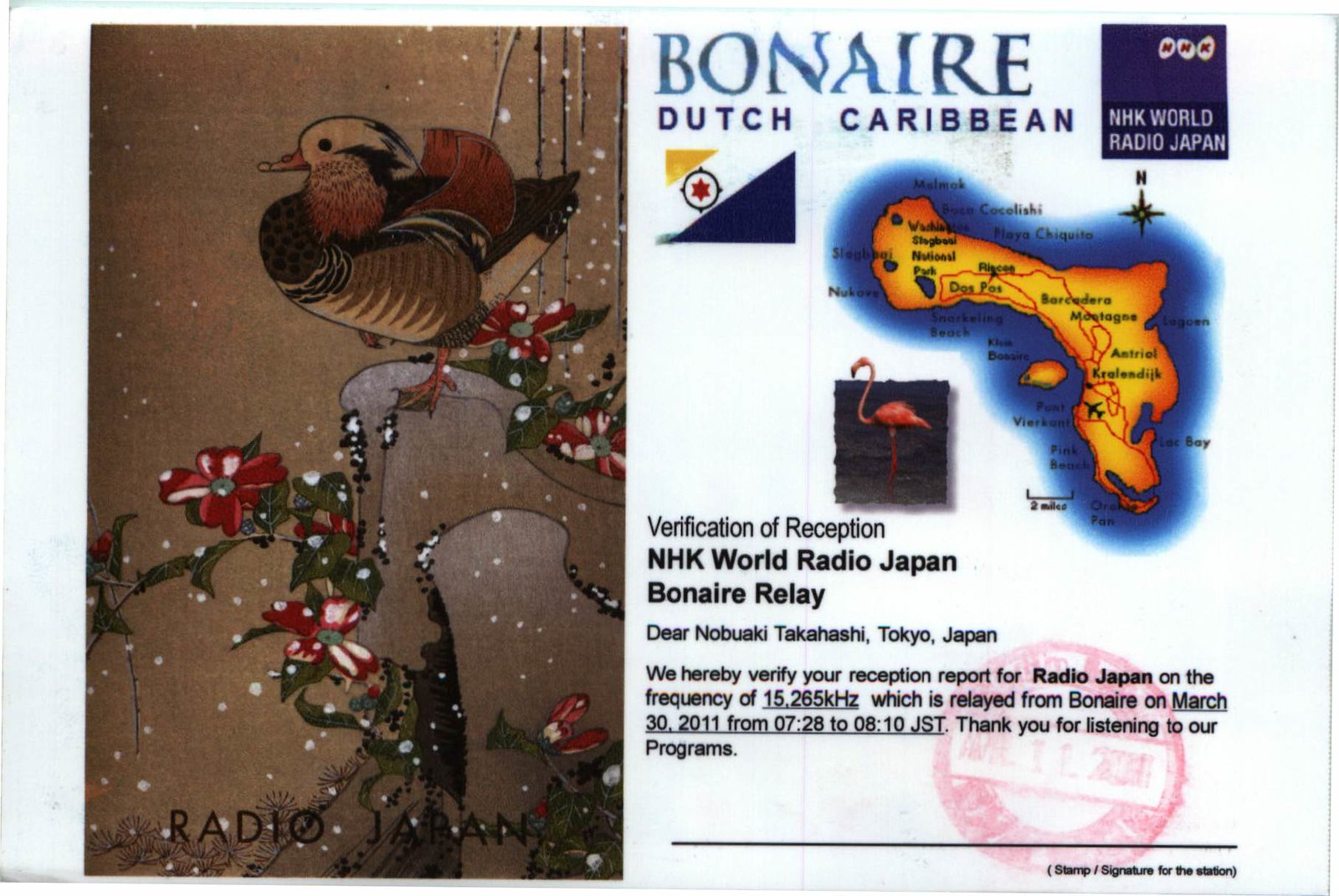This image depicts a receipt-like postcard divided into two vertical sections. The left third features an illustration of a multi-colored duck on a snowy embankment surrounded by red flowers with green leaves. Below this is the text "Radio Japan" in black font. The right two-thirds is dominated by detailed text that starts with the header "Bonaire, Dutch Caribbean" and includes a depiction of the Bonaire flag, which features a yellow triangle, a white center with a black circle and red star, and a dark blue triangle. Below the flag is a schematic map of Bonaire with various locations labeled, such as Malmo, Playa Chiquita, and Dos Pos, among others. Adjacent to the map is an image of a flamingo standing on water. Underneath this is black text that reads: "Verification of Reception, NHK World Radio Japan, Bonaire Relay. Dear Nobuaki Takahashi, Tokyo, Japan, we hereby verify your reception report for Radio Japan on the frequency of 15.265 kHz, which is relayed from Bonaire on March 30, 2011, from 7:28 to 8:10 JST. Thank you for listening to our programs." A watermark logo and a stamp or signature appear at the bottom right corner.